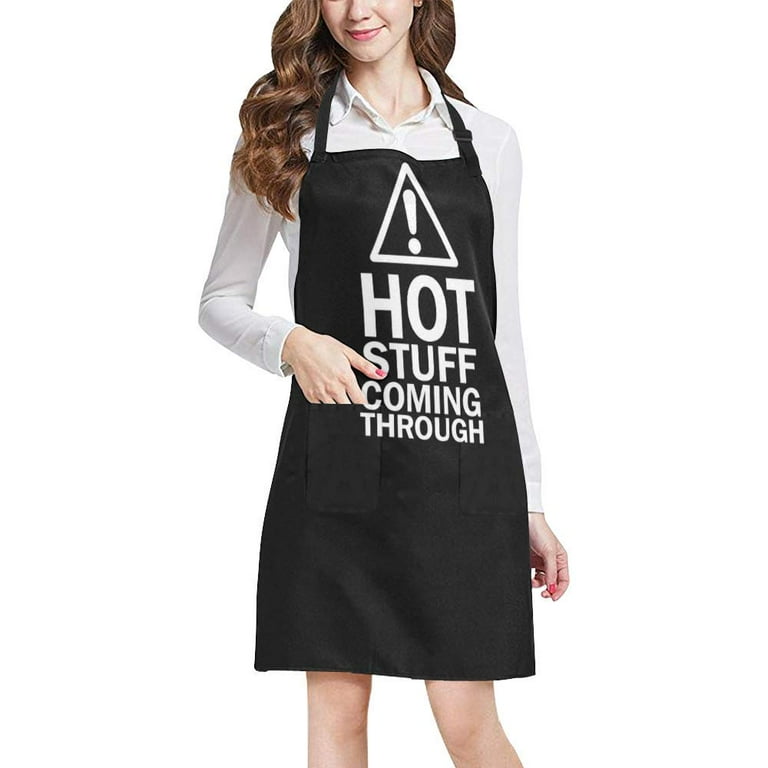The photograph features a young woman modeled against a white background, captured from just below her nose to the bottom of her knees. She has long, brown hair and is wearing a crisp, white, long-sleeved, button-up shirt with an open collar. Over her shirt, she dons a knee-length, black apron that prominently displays a white, upside-down triangle with an exclamation mark in the center. Below the triangle, the text "HOT STUFF COMING THROUGH" is emblazoned in white, with "HOT" in particularly large letters. Her left hand has a few fingers casually tucked into a pocket of the apron, while her right arm hangs naturally by her waist, showcasing red nail polish. The image is professionally captured, resembling a product display commonly seen on e-commerce websites like Amazon, and the model's relaxed pose and slight smile effectively highlight the apron.